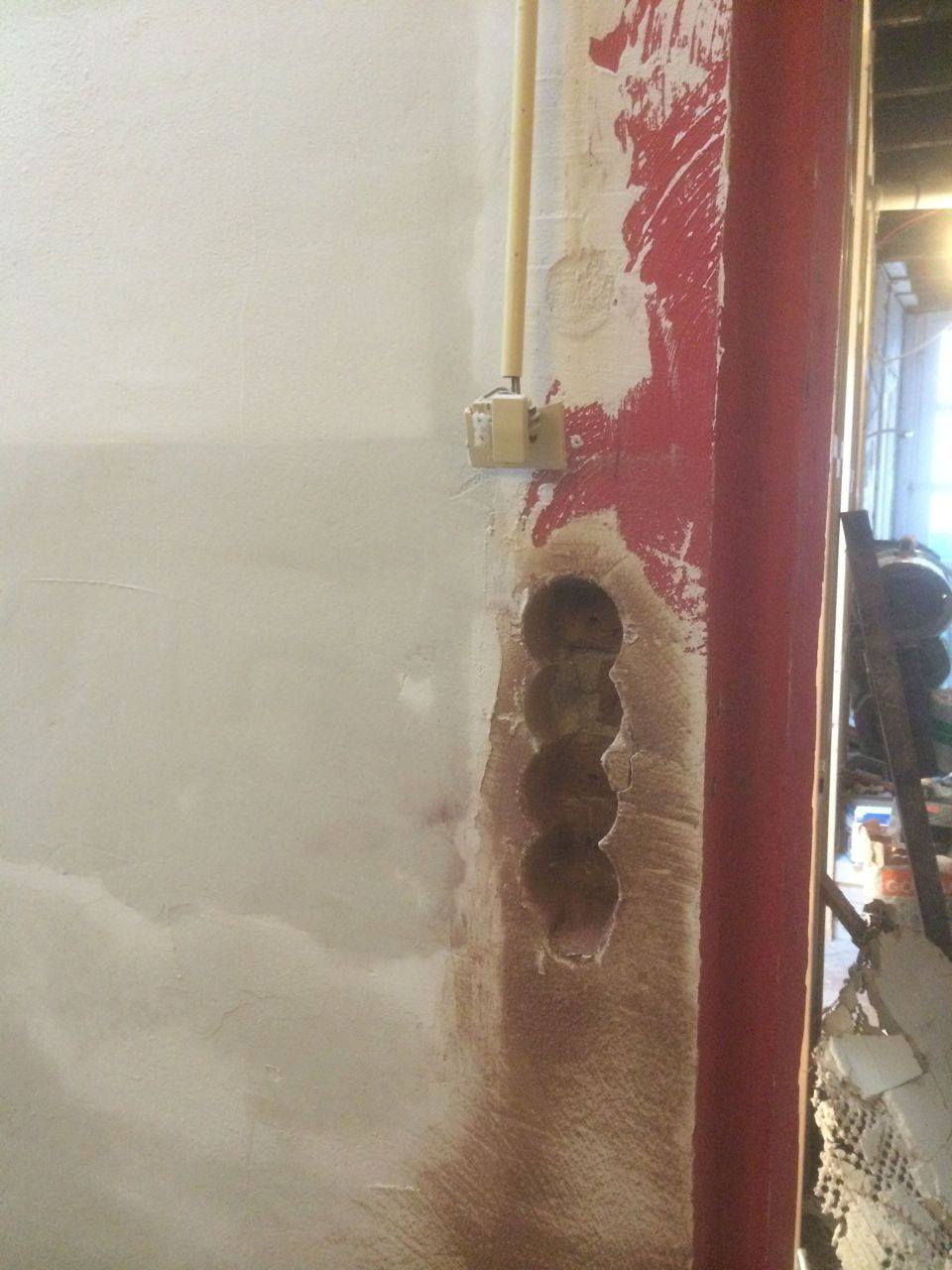The photograph captures an unfinished wall in an interior construction zone, dominated by distinct construction features. Centrally, four overlapping circular indentations forming a vertical slot are clearly visible, resembling stacked tin can imprints. The wall is predominantly light-colored plaster with a darker brown hue surrounding the holes. Above the indentations, an area is coated with red paint, which seems to have been haphazardly applied. A piece of plastic conduit ascends the wall from the center, housing electrical cables, possibly leading to a socket or telephone outlet. The right corner of the image reveals additional construction materials, including a bucket and broken plaster pieces, illuminated by both an unfinished ceiling light and natural light from an open window. The combined elements suggest an ongoing construction project, with various stages of completion and exposed building components.